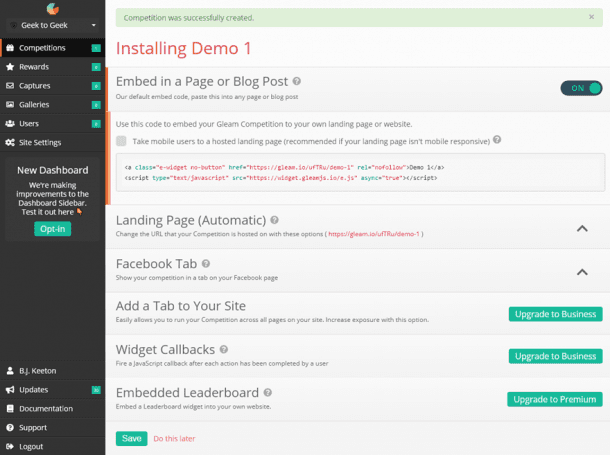Sure, here is a cleaned-up and detailed caption for the described image:

---

The image showcases the "Geek2Geek" website interface. On the left side of the screen, there is a sleek, black vertical menu with options listed in white text. The menu items include: Geek2Geek, Competitors, Rewards, Captures, Galleries, Users, Site Settings, and New Dashboard. Beneath these, a section highlights ongoing improvements with the text: "We're making improvements to the dashboard sidebar. Test it out here," followed by a green "Opt-in" button. At the very bottom of the menu, the text reads: "BJ Keaton, Updates, Documentation, Support, Logout."

In the main content area of the screen, a notification confirms: "Competition was successfully created." Additional instructions follow, detailing the process for embedding the competition into a page or blog post. It reads: "Install Demo One. Embed this into any page or blog post using our default embed code. Use this code to enable your Gleam competition on your own landing page and website. Direct mobile users to a hosted landing page, recommended if your landing page isn’t mobile responsive."

Below these instructions, an embedding code is displayed along with several additional options: "Landing Page Automatic, Facebook Tab, Add a Tab to Your Site, Widget Callbacks, Embedded Leaderboard." Users are prompted to "Save" or choose to "Do this later." The visual elements on the page feature a mix of green, red, gray, black, and white colors.

---